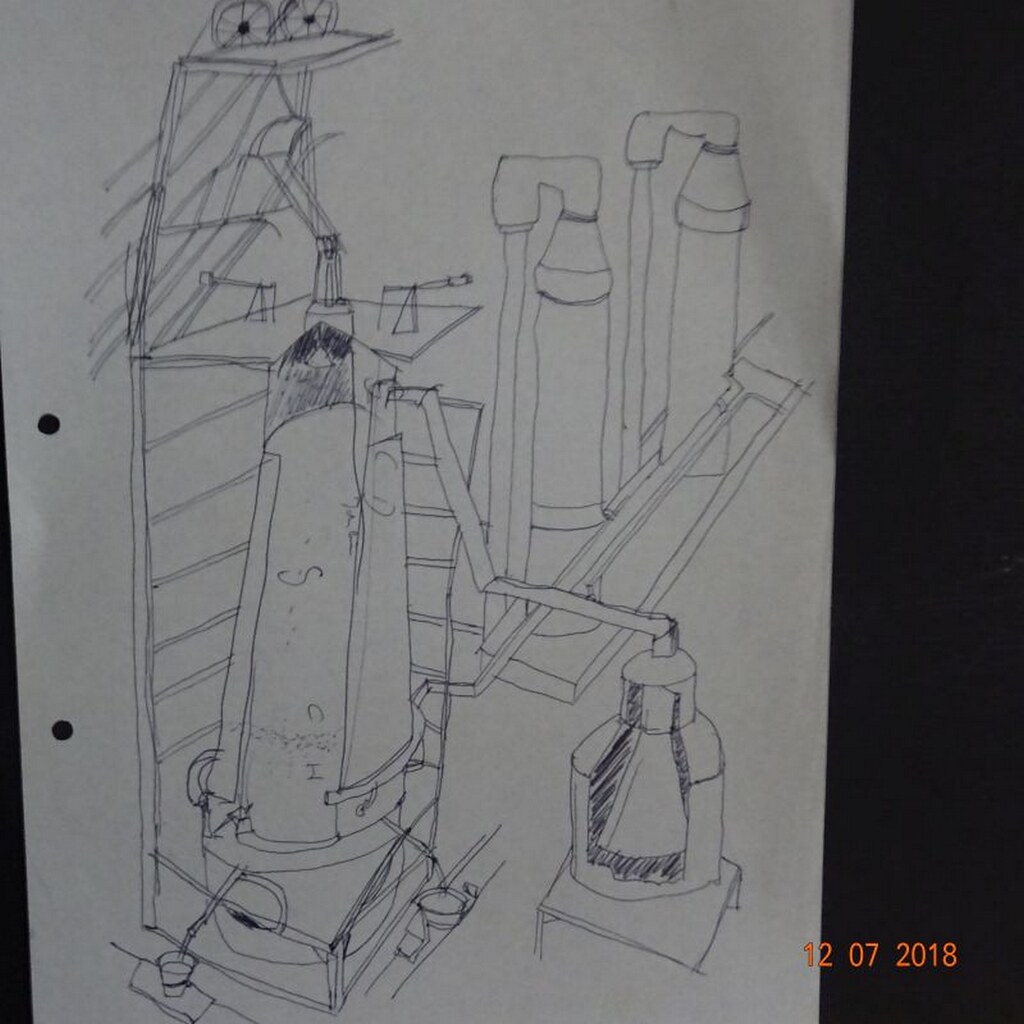The image features a child's drawing on a standard sheet of white paper, which has two holes punched on its left side. The paper is set against a dark black background. In the bottom right-hand corner, the date "12-07-2018" is written in orange. The drawing itself, sketched in pencil or pen, depicts a complex, industrial-like scene with interconnected components. There are several units resembling boilers or mechanical structures, including what appear to be holding containers or vats labeled with the letters C, D, S, C, and I. These elements are interconnected with tubes, wires, and railings, creating an intricate and somewhat ambiguous depiction of a factory or mechanical setup.